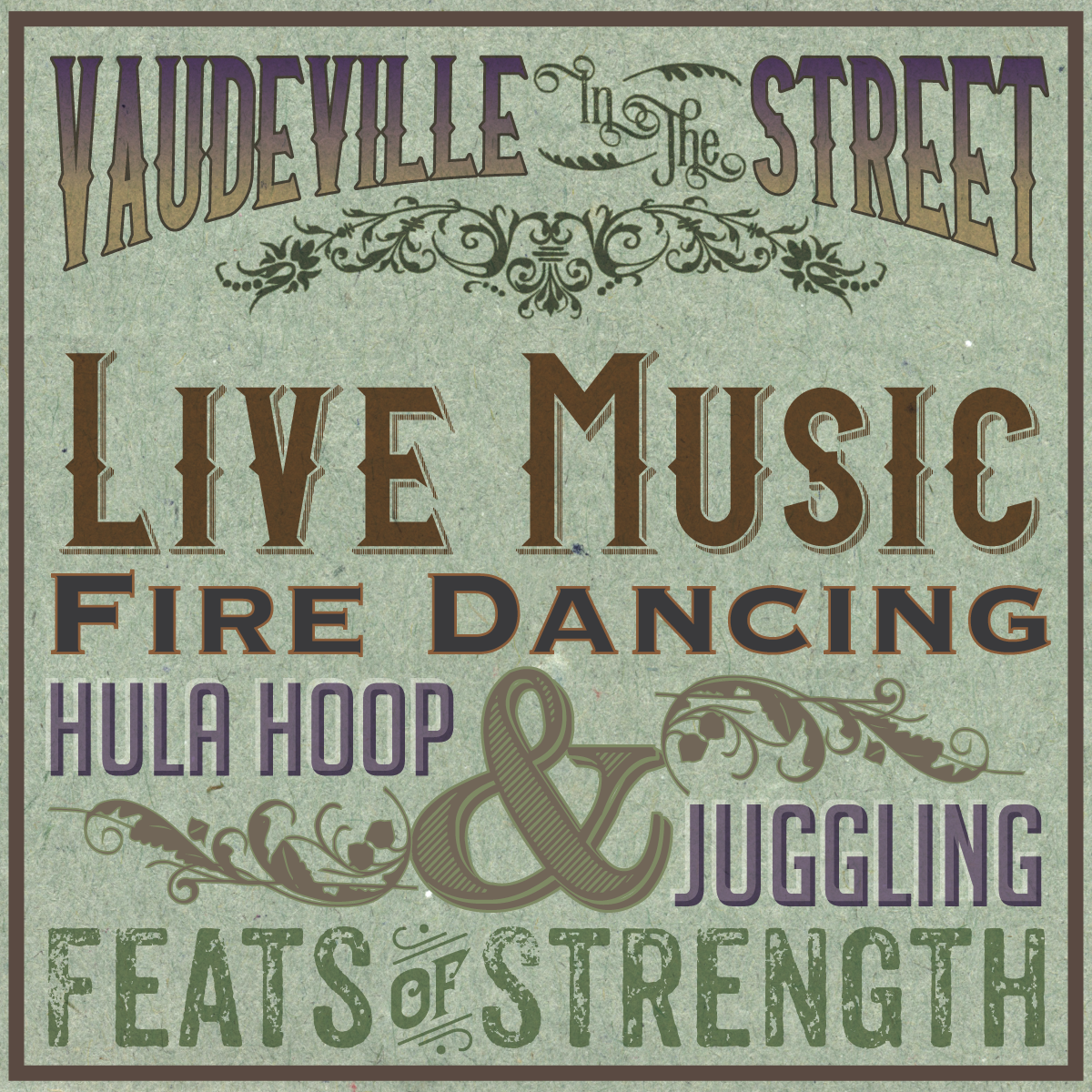This square poster, designed to evoke an old tin sign, promotes an event with a rustic, vintage flair. The textured background is a blend of light green and gray, reminiscent of worn, old-style imagery. Framed by a thin dark brown border, the top of the poster features the phrase "Vaudeville in the Street" in an ornate, old-school font. Below it, the event highlights are listed in five lines, each in a distinct style and color to enhance the eclectic vibe: "Live Music" in brown, "Fire Dancing" in dark gray, "Hula Hoop" in purple, "Juggling" with a prominent 'and' symbol, and "Feats of Strength" in a stamped, olive-green font. Interspersed with vine-like decorative elements, the text adopts various serif and sans serif fonts, primarily in shades of brown, but also featuring pops of purple, blue, orange, and green, encapsulating a whimsical, vaudevillian theme.